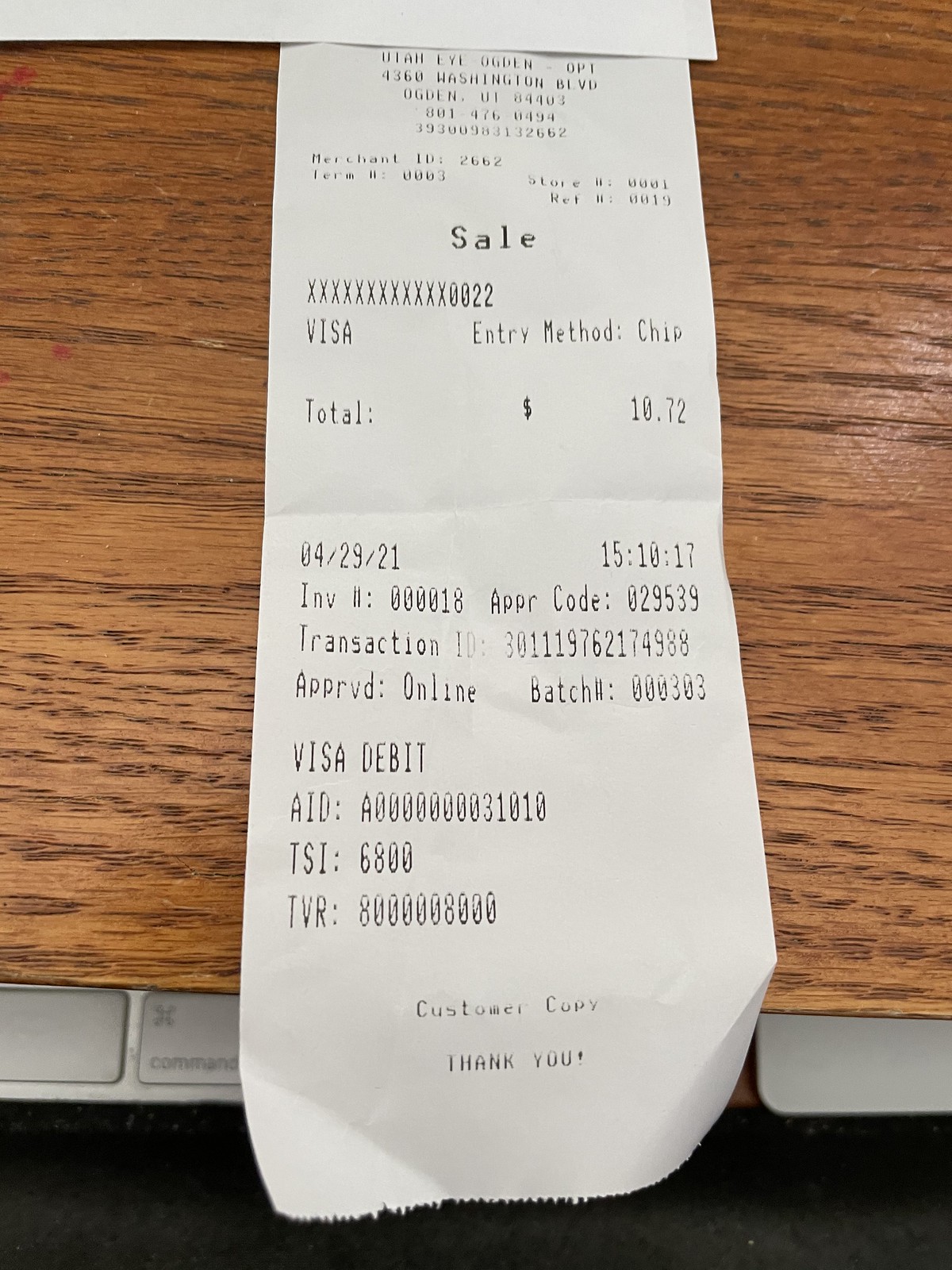The image depicts a slightly faded, white receipt from a store identified as "UtahIOgden.opt," located at 360 Washington Boulevard, Ogden, Utah, 84403. The receipt is placed on a light to medium brown table or desk, possibly faux wood, and a black keyboard key with the word "Command" is visible at the bottom left of the frame. The receipt details a transaction made with a Visa debit card using the chip entry method. Notable information includes the Merchant ID: 2662, Terminal: 0003, Store Number: 0001, and Reference Number: 0019. The total amount of the purchase is $10.72, and the transaction occurred on April 29, 2021, at 15:10:17. Additional transaction details include an Invoice: 0000018, Approval Code: 029539, Transaction ID: 301119762174988, the batch number: 000303, and the identifiers AID: A0000000031010, TSI: 6800, and TVR: 8000008000. The document concludes with the note "Customer Copy" and a "Thank You" message at the bottom.